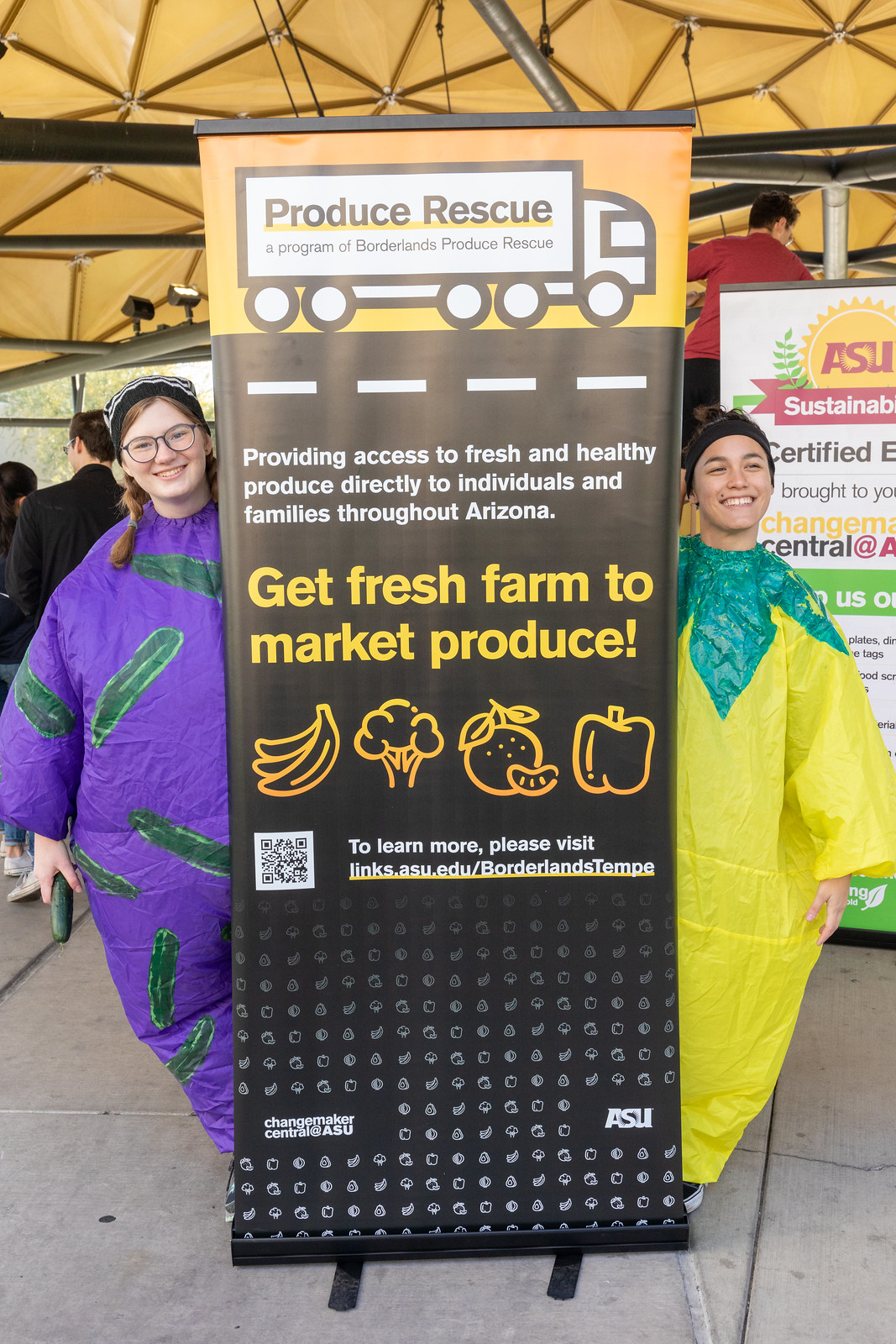In this color daylight photograph taken under a yellow pavilion-like tent supported by black beams, we see two women dressed in quirky inflatable outfits, posing beside an upright sign. To the left, the woman with fair skin and light brown hair, sporting dark-framed glasses, a black handkerchief, and braids, smiles while holding a cucumber. She wears a purple suit adorned with cucumbers. On the right, her companion in a yellow outfit with greenish teal shapes and a black headband similarly smiles at the camera. Both women are cheerful and engaged in their promotional task.

The central sign they lean from behind prominently displays "Produce Rescue" with a drawing of a semi-truck at the top. Below the truck, text highlights "Providing access to fresh and healthy produce directly to individuals and families throughout Arizona." Further down, in bold yellow letters, "Get Fresh Farm to Market Produce" is followed by stylized drawings of bananas, broccoli, an orange, and a pepper. Additional information, including a QR code and the website "links.asu.edu/BorderlandsTempe," is provided in smaller white text at the bottom, alongside logos for Changemaker Central and ASU. The sign stands on black feet on a concrete floor, while background details reveal more signs and people, enhancing the lively atmosphere of this market event.